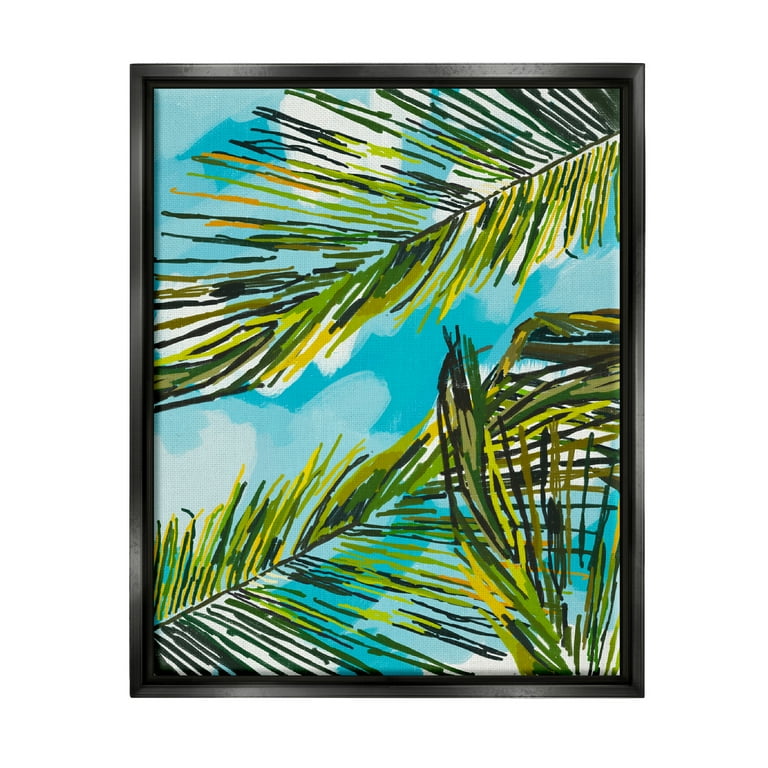This artwork is a framed painting or illustration featuring at least three large, fern-like palm leaves, characterized by their fine, needle-like sections branching off a middle stem. The leaves are depicted in varied hues of green, yellow, dark green, light green, gray, and touches of gold, blending harmoniously. The background is adorned with splotches of blue that represent the sky, interspersed with different shades and shapes of white clouds, creating a dynamic atmosphere. The frame itself appears to be a slender, angular wooden design, dark brown or charcoal in color, adding a refined touch to the modern artwork. The painting has a somewhat child-like or whimsical style, yet exudes a sense of modern artistic flair.